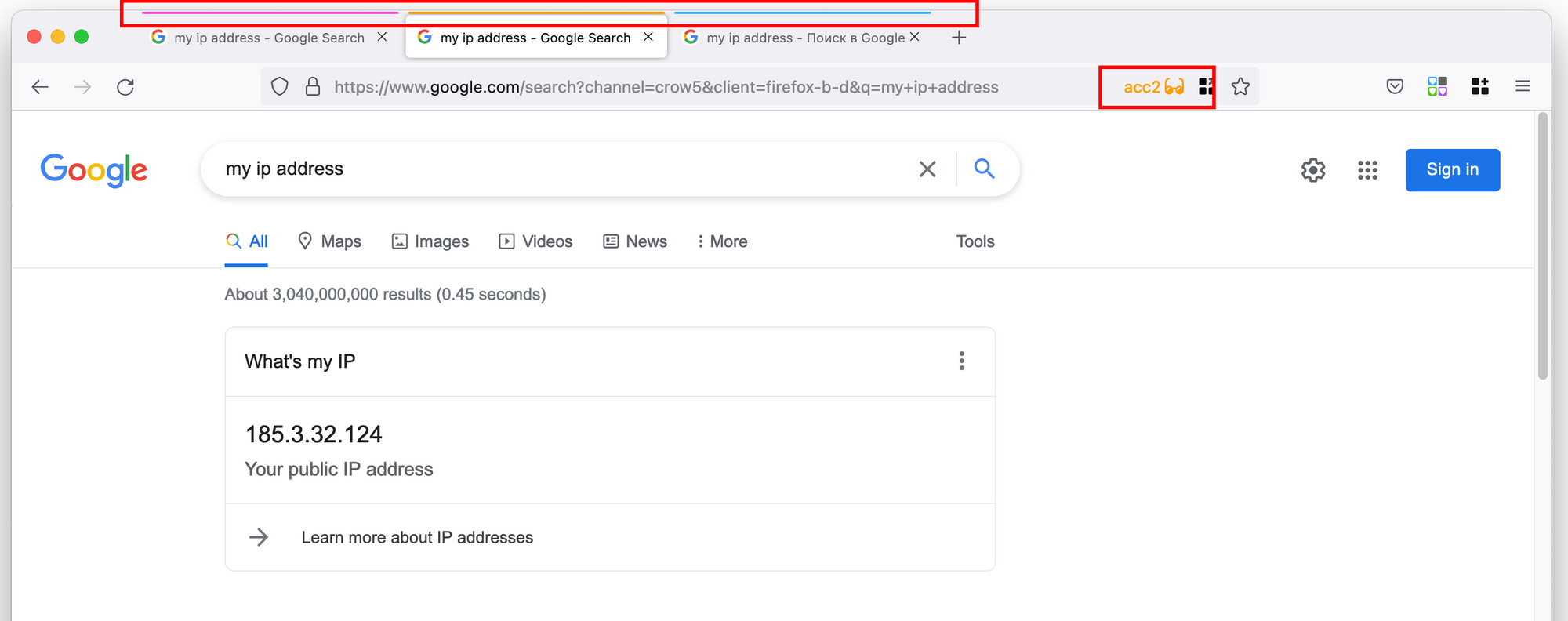A detailed caption for the given image description:

---

A screenshot of a Chromebook displaying a web browser with three open tabs in the far left corner, each adorned with a red, yellow, and green circle for window controls. The browser is in Google Chrome with three tabs open. The first tab shows the Google logo and reads "my IP address / Google search," with a close button (X) beside it. The second tab, currently selected, also shows "my IP address / Google search." The third tab features "my IP address" followed by Russian Cyrillic script, and there is a plus (+) symbol for adding a new tab.

Below the tabs, the browser's toolbar displays a back arrow, a grayed-out forward arrow, and a reload button. To the right, there is a secure lock icon indicating a secure connection, followed by the URL "https://www.google.com/search?channel=crow5". Also visible are extensions or browser add-ons: a shielded checkmark icon, two four-pane icons, one with varying color panels (blue, green, pink, and black) and another fully black. Further right is a menu button represented by three horizontal bars.

The main browser window shows the Google logo on the far left, and beside it, a search bar with the query "my IP address" in black lowercase text. There is a close (X) button and a magnifying glass icon beside the search query. Below the search bar, a banner displays the IP address "185.3.32.124" labeled as "Your public IP address." To the right, there is a blue hyperlink "Learn more about IP addresses" with an arrow pointing right. The browser appears in day mode with a white background.